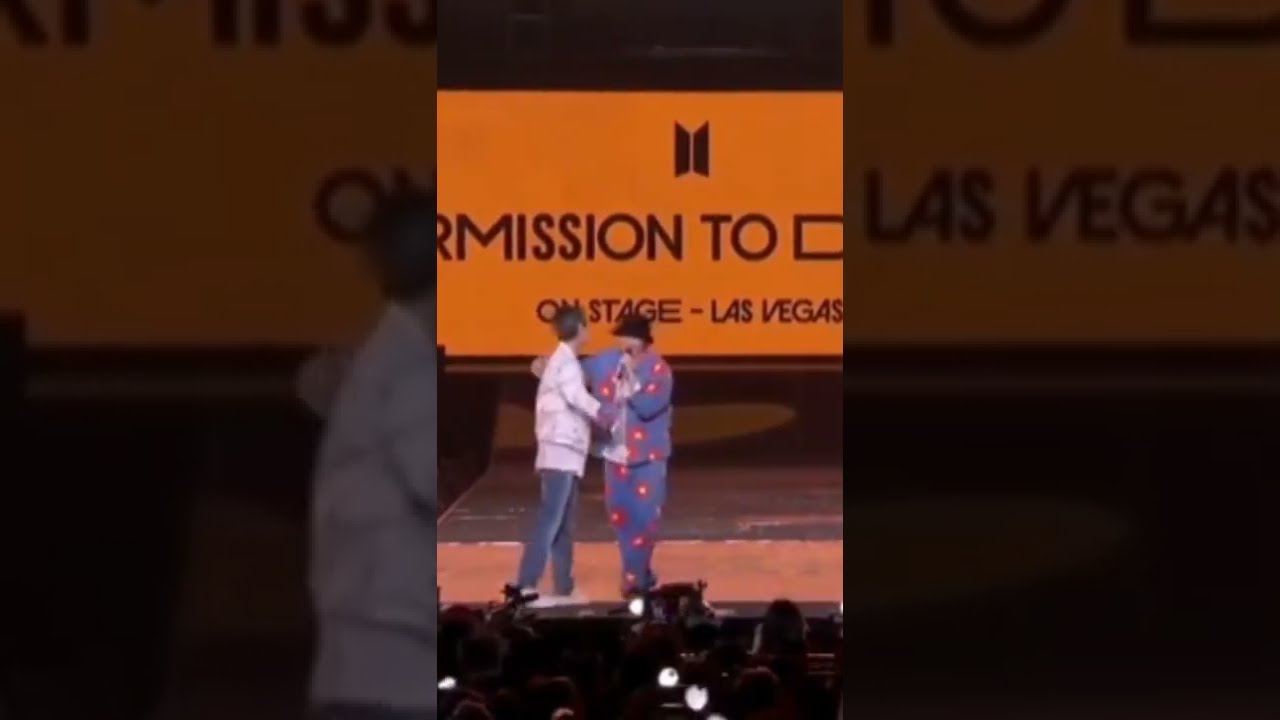The image depicts a vibrant live stage event, set against an orange backdrop adorned with partially visible black text that appears to read "Mission 2" and "On Stage Las Vegas." Central to the composition are two individuals embracing. The man on the right is dressed in a striking blue outfit, featuring matching pants and a jacket embellished with red circles and bright orange centers. He wears a black hat reminiscent of a bowler hat and holds a black microphone close to his face. The individual on the left sports a white long-sleeve shirt and either gray or blue pants. Their attire contrasts subtly with black footwear that resembles clogs. Below the stage, an engaged audience captures the moment on their cell phones, adding to the lively atmosphere. The overall scene is layered with a darker, zoomed-in version of itself, enhancing the focus on the central figures and creating a vivid, dynamic visual effect.